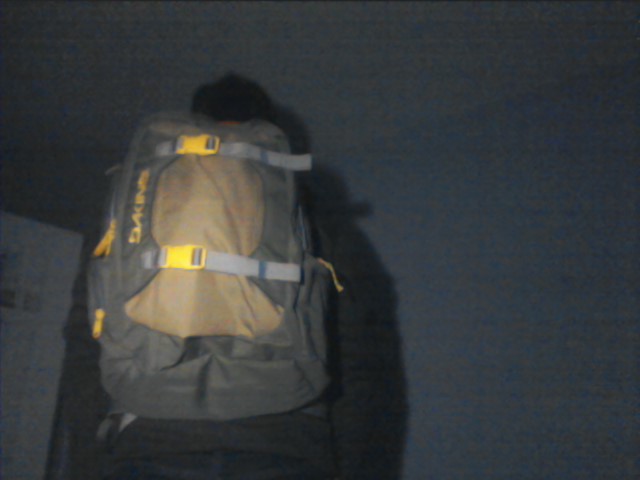The image depicts a dimly lit, indoor setting, possibly a living room at night. The background features shades of gray, black, yellow, brown, orange, white, and bluish-gray, creating a somewhat dark and muted atmosphere. On the left side of the image, a white door is visible, likely the front door of the house. The focal point of the image is a man standing near the center, dressed in warm, dark clothing including a gray long-sleeve sweatshirt or jacket and dark pants. He has a backpack on his back, which is gray with yellow lettering on the left side, possibly spelling "DAK," and equipped with gray straps that have yellow buckles. The man's hair is black, and he is facing away from the camera, with a faint shadow cast to the right of his head. The overall image is slightly blurry but richly colored, enhancing the dim, nighttime ambiance of the scene.